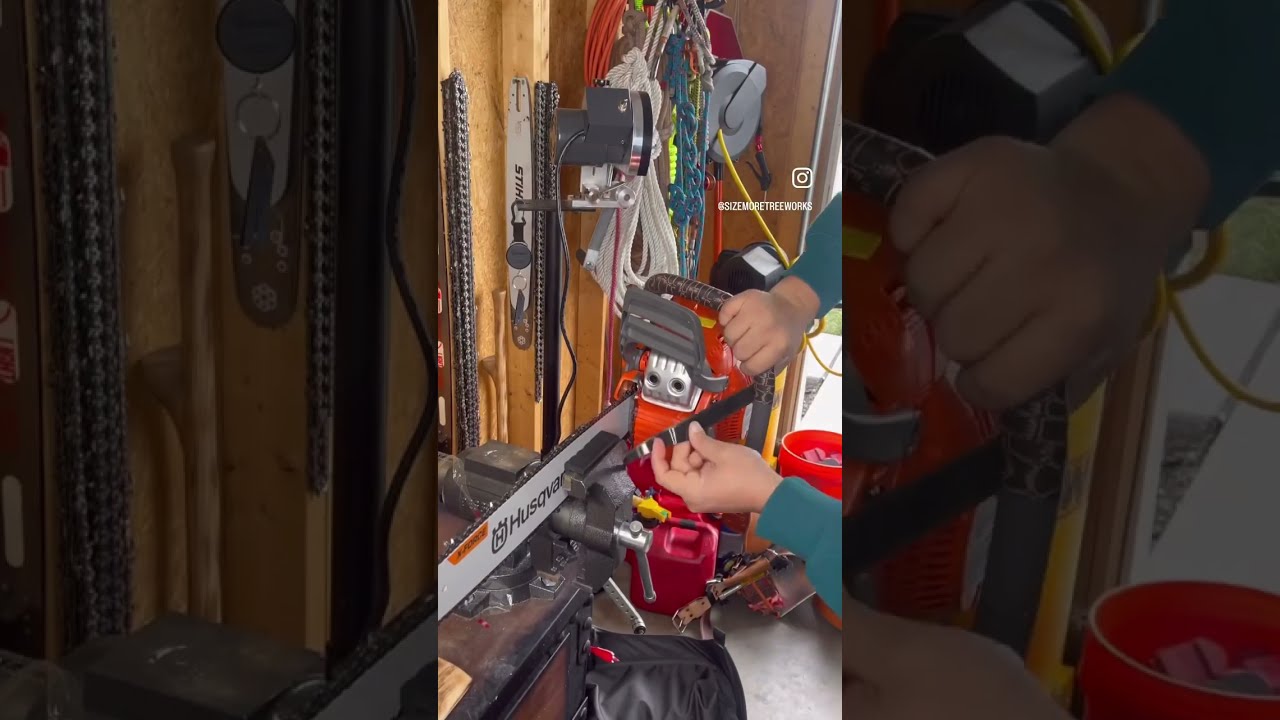The image is a vertically oriented photograph with a zoomed-in, darkened filter overlay and the full, naturally lit picture spliced into its center. The main scene depicts an unfinished garage with exposed wood framing and various tools and equipment hanging on the walls. Visible in the background are an assortment of chains, pulleys, ropes, and extension cords neatly looped and hung. A brown-skinned individual wearing a dark green long-sleeved shirt is prominently holding a Husqvarna chainsaw, whose blade extends out of the left edge of the image. The body of the chainsaw is orange, and its handle area is gray, with the blade featuring a black edge. The person appears to be working on the chainsaw, possibly reattaching or sharpening the chain while holding it in a vice grip. Additional details include a bucket of parts and various other items such as saws, measuring tapes, and a gasoline can scattered throughout the workspace. The overall scene is set inside what appears to be a tool shed or garage, characterized by natural daylight streaming in through an open garage door. A small camera symbol is visible in the top right corner, suggesting the photo might be from a social media video platform like Instagram.